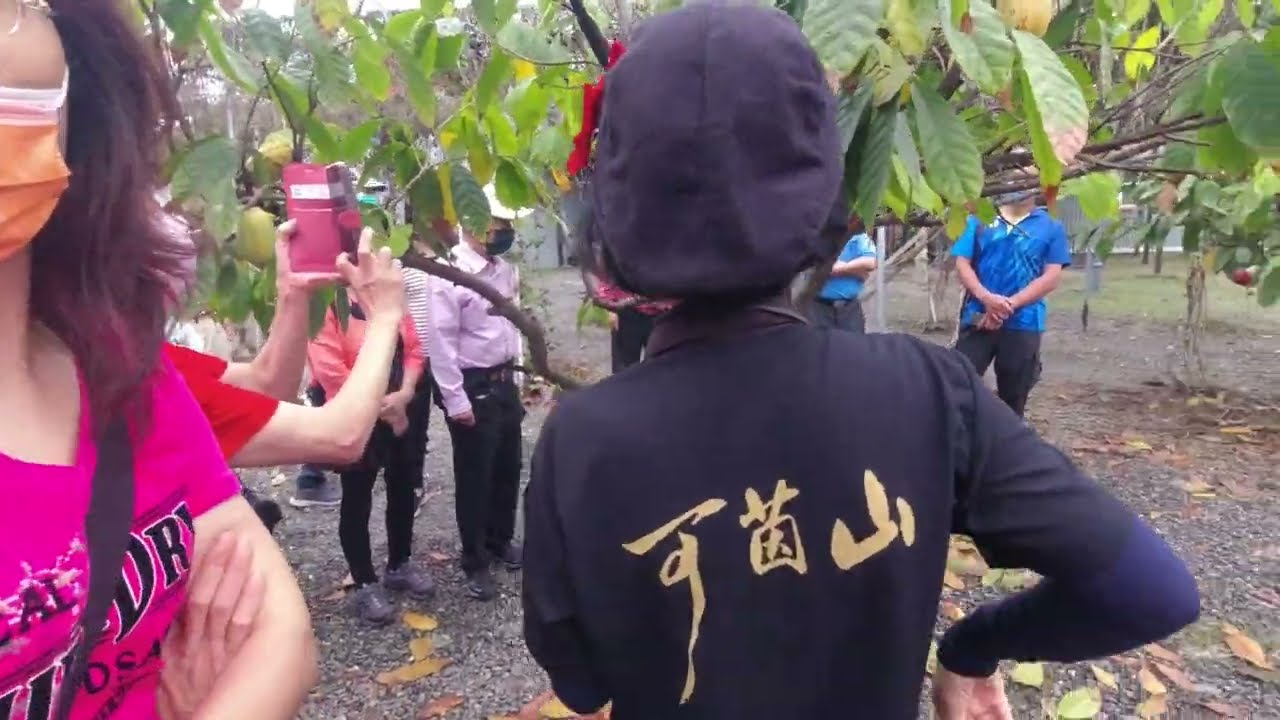The horizontally aligned rectangular outdoor image captures a group of people gathered around a central tree with low-hanging branches and abundant leaves. Dominating the foreground, the back of an ambiguous person — possibly male or female — is seen wearing a backwards black beret and a dark blue long-sleeve shirt adorned with gold symbols reminiscent of Asian characters. To the left, a partially visible woman with shoulder-length brown hair, wearing a dark pink shirt with black writing and an orange and white mask, is present. Another individual behind her, clad in a red short-sleeve shirt, holds up a pink rectangular object. Further to the right, partially obscured by tree branches, stands a person in a blue short-sleeve shirt and black pants. The ground is gravelly, scattered with fallen leaves, and a building is faintly visible through the foliage in the background.